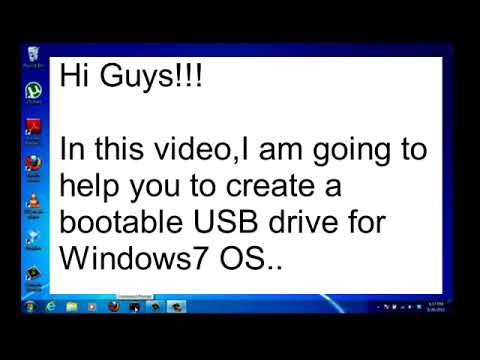This image is a detailed screenshot of a Windows computer home screen, seemingly from an older version of the Windows operating system. At its core, it is a step-by-step visual guide on how to run the Command Prompt (CMD) as an administrator. The main section of the screen displays a Windows interface with the iconic logo in blue at the center, showcasing the familiar yellow, green, red, and blue wave flag. White text on a black rectangle in the upper-left corner states, "1. Run CMD command as administrator," indicating the first step in the process.

In the bottom left corner, the Start menu is open, with the search bar populated with the text "CMD." A gray rectangular context menu appears, displaying options for interacting with the application. The arrow cursor hovers over the "Run as administrator" option, highlighting it, suggesting the imminent selection of this command.

Throughout the screenshot, various common elements of the Windows interface are visible, including the Internet Explorer and Firefox icons, as well as system tray icons for Wi-Fi, sound, and the clock. Adobe and possibly other icons are obscured partially by the black rectangle and border encasing the entire image. This detailed walkthrough is designed to guide users through the process of opening the command tool with administrative privileges in older Windows versions.